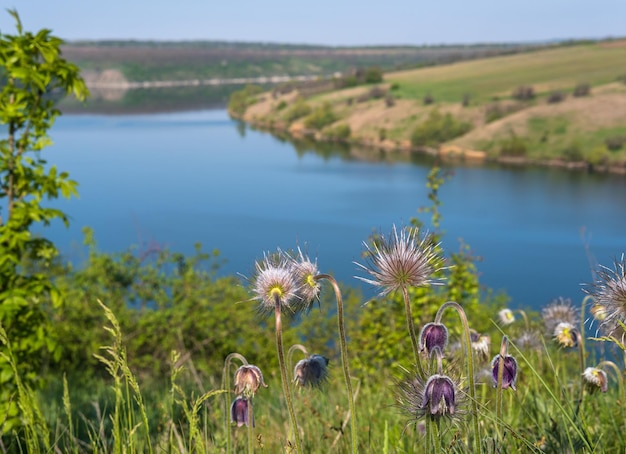In this vivid photograph of a serene outdoor nature scene, the focus is on an up-close section of a tranquil lake with bright bluish water, bordered by a rich tapestry of colorful flowers and vegetation. The foreground is filled with tall green grasses interspersed with various blossoms, predominantly in shades of purple, pink, and white, many of which have spiked heads or are slightly drooping. To the left, a prominent tree adds to the lush greenery, while the top right reveals a gently downsloping hill covered in green bushes and grass, leading directly into the lake. The image captures the essence of a bright, sunny day, as indicated by the clear blue sky spreading above and the vivid sunlight illuminating the flora and water below. In the distant backdrop, the landscape transitions into more green vegetation with sporadic patches of barren dirt and possible thickets or trees, all adding depth to this peaceful and beautifully detailed nature setting.